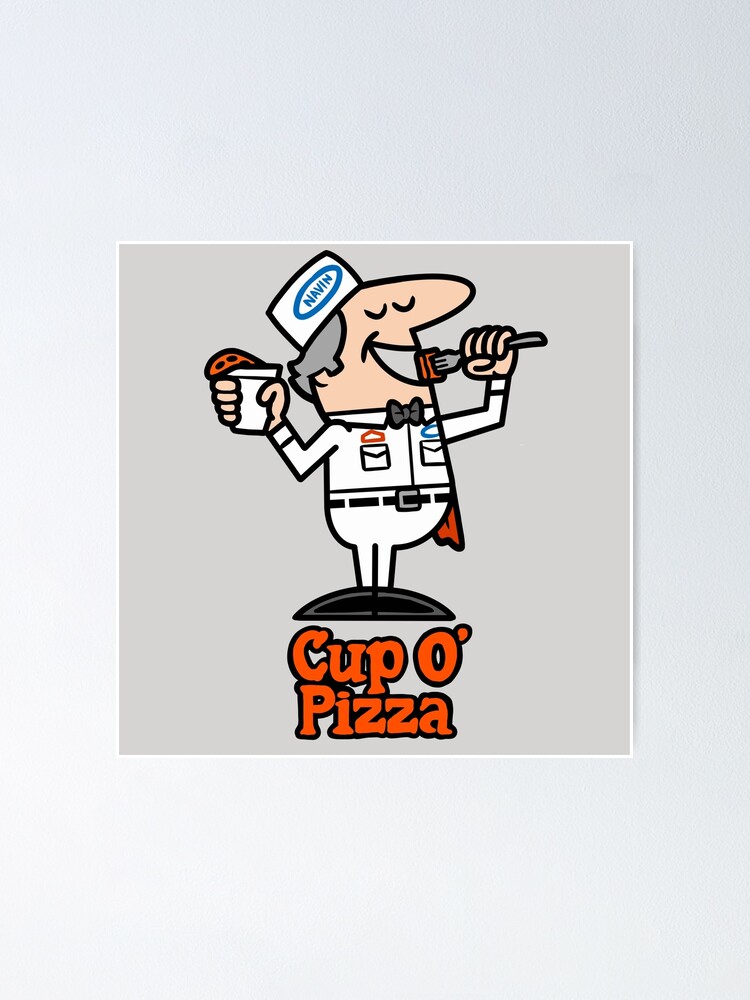A cartoon figure dressed in a crisp white uniform with a dogged line belt is holding a small white cup in their right hand. Emanating from the top of the cup is a tongue-like brown substance. The figure wears a white cap inscribed with the letters "M-A-B-I-N" in blue, encircled in blue. Below the figure, the words "Cup-O-Pizza" are prominently displayed in orange. In their left hand, the figure grips a fork, which is spearing a square piece of reddish-brown food. The uniform features two envelope-like pockets: the left pocket is adorned with an oddly-shaped, five-sided orange design, while the right pocket displays a blue circle.